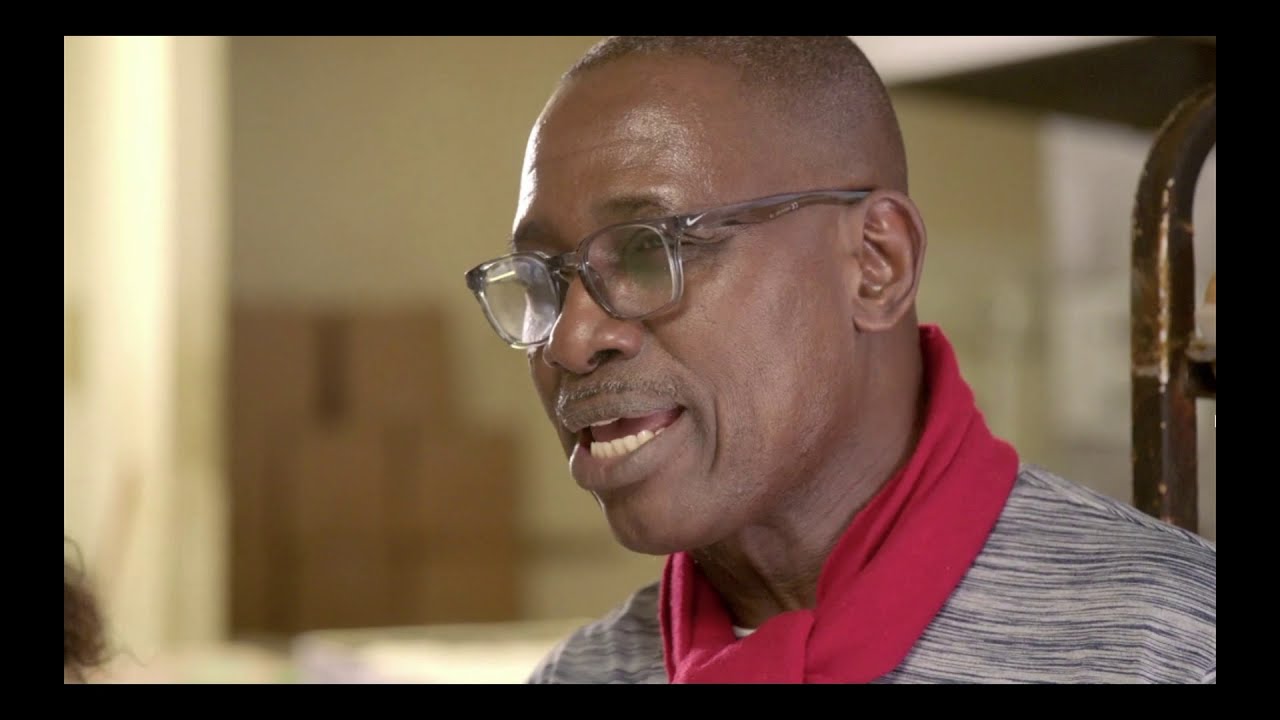This landscape color photograph, measuring approximately eight inches wide by five inches tall, is framed by a quarter-inch thick black border. It features an elderly African-American man, possibly in his 60s, with closely trimmed hair and a mustache. He is photographed mid-speech, with his mouth open, revealing his teeth and tongue. His face is angled slightly to the side, almost in profile, allowing a clear view of his expression.

The man is wearing translucent, smoky gray eyeglasses adorned with the white Nike swoosh logo on the side. His attire includes a black and white striped shirt and a thin red sweater, preppy-style, tied around his neck. His dark brown skin tone is highlighted, and his accessories, particularly the glasses, contribute to the detailed characterization.

In the background, which is noticeably out-of-focus, there is a beige wall with a stack of cardboard boxes, approximately three boxes high. To the right of the man is some kind of metal shelving or structure with peeling paint. A white upright column is visible to his left. These background elements, although blurred, add to the contextual setting of the photograph.